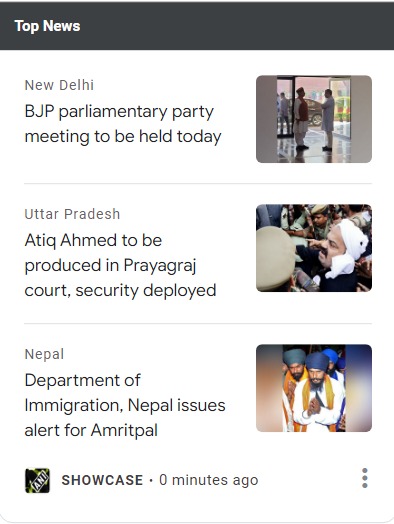The image depicts a segment of a news website. The top of the image features a dark gray background with prominent white text reading "Top News." Directly below, the layout transitions to a white background divided into three distinct sections:

1. **New Delhi**: The headline announces, "BJP Parliamentary Party meeting to be held today," accompanied by an image on the right showing two individuals engaged in a meeting.
 
2. **Uttar Pradesh**: The section highlights, "Fatik Ahmed to be produced in Prayagraj court, security deployed," with a relevant image illustrating the description.

3. **Nepal**: The final segment alerts, "Department of Immigration, Nepal issues alert for Amritsarpal," featuring an image of Amritsarpal with two men standing behind him.

At the bottom, the words “Showcase” are visible, noted as being updated "zero minutes ago," with a trio of small dots situated at the bottom right of the image.